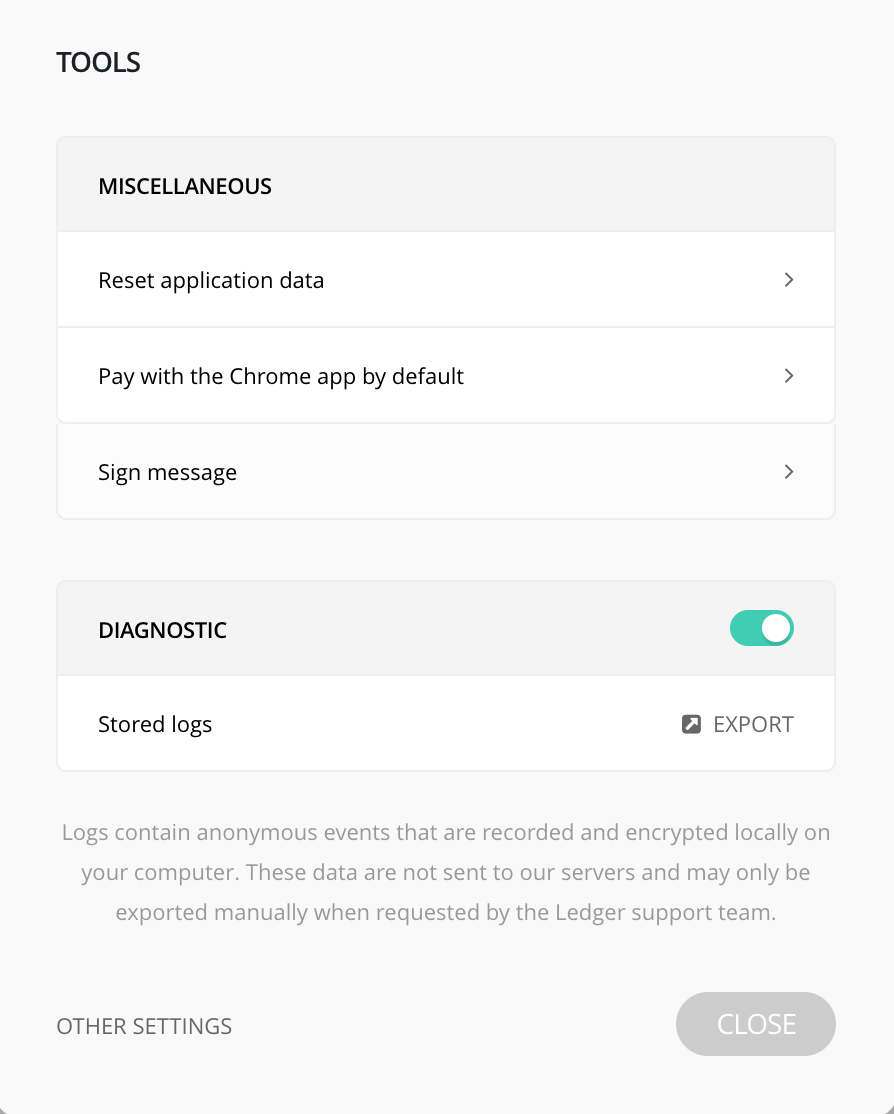The image is a screenshot of a settings menu with a white background, containing several segments and options with varying shades of gray and accents of teal. 

In the upper left corner, the word "TOOLS" is prominently displayed in bold, black, capital letters on a slightly different white background than the rest of the image. Below "TOOLS," the word "MISCELLANEOUS" appears, also in black, capital letters.

Further down, there is a horizontally elongated white strip containing the text "RESET APPLICATION DATA" in black. To the right of this text, there is a right arrow icon. 

A gray line separates this section from the next, where "PAY WITH CHROME APP BY DEFAULT" is written in black with another right arrow icon to the right. 

Below another gray line, the text "SIGN MESSAGE" appears, accompanied by another right arrow icon on its right side. 

Proceeding further down, the word "DIAGNOSTIC" is displayed in black, capital letters, next to a teal toggle switch, which is currently turned on. 

Below the toggle switch, on another white background, the text "STORED LOGS" is visible with an "EXPORT" button to its right. Underneath this, a more detailed explanation states: "Logs contain anonymous events that are recorded and encrypted locally on your computer. These data are not sent to our servers and may only be exported manually when requested by the Ledger support team."

At the bottom left corner, "OTHER SETTINGS" is written in black, capital letters. On the right side of this text, there is a gray button labeled "CLOSE" in white font. 

The overall color scheme features shades of black, gray, white, and teal, with variations from very pale gray to slightly darker gray.